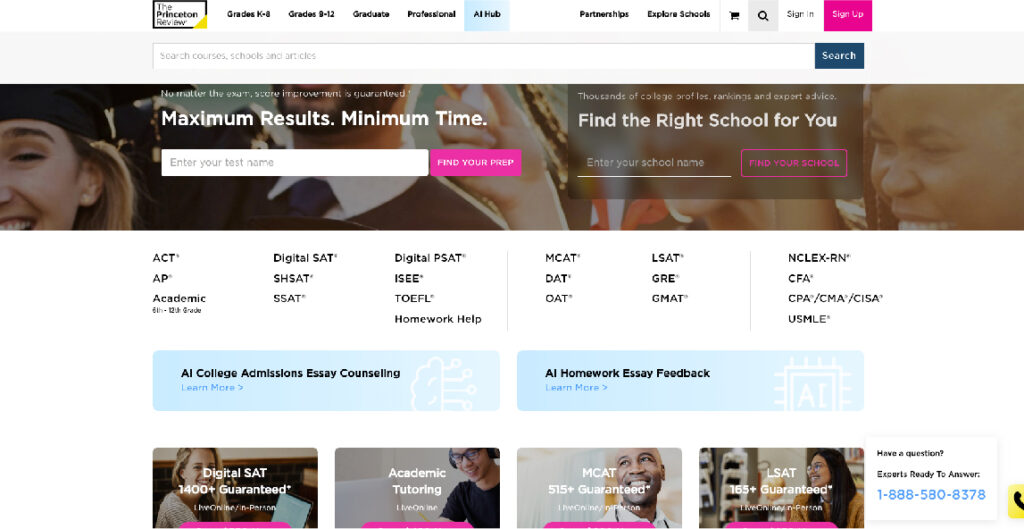The image showcases a detailed view of the Princeton Review website. The background is predominantly white, exuding a clean and professional appearance. At the top of the page, several navigational tabs are neatly arranged, including "Grades K-8," "Grades 9-12," "Graduate," "Professional," "AI Hub," "Partnerships," and "Explore Schools." The Princeton Review's logo is displayed prominently in a black and white box at the upper left corner.

To the right of these tabs, icons for a shopping cart and a search function are visible, along with "Sign In" and "Sign Up" buttons, providing quick access to user accounts. Below these elements, a search bar with a blue button invites users to explore further.

The central header features an image of students celebrating graduation, capturing a moment of academic achievement. Below the image, there are two primary call-to-action sections: "Find Your Prep" with a corresponding button, and "Find the Right School for You," positioning the website as a resource for educational advancement.

Further down, the site provides additional informational sections, including AI-based services such as "AI College Admission," "Essay Counseling," and "AI Homework Essay Feedback." Underneath these offerings, more navigational tabs direct users to various other resources available on the website.